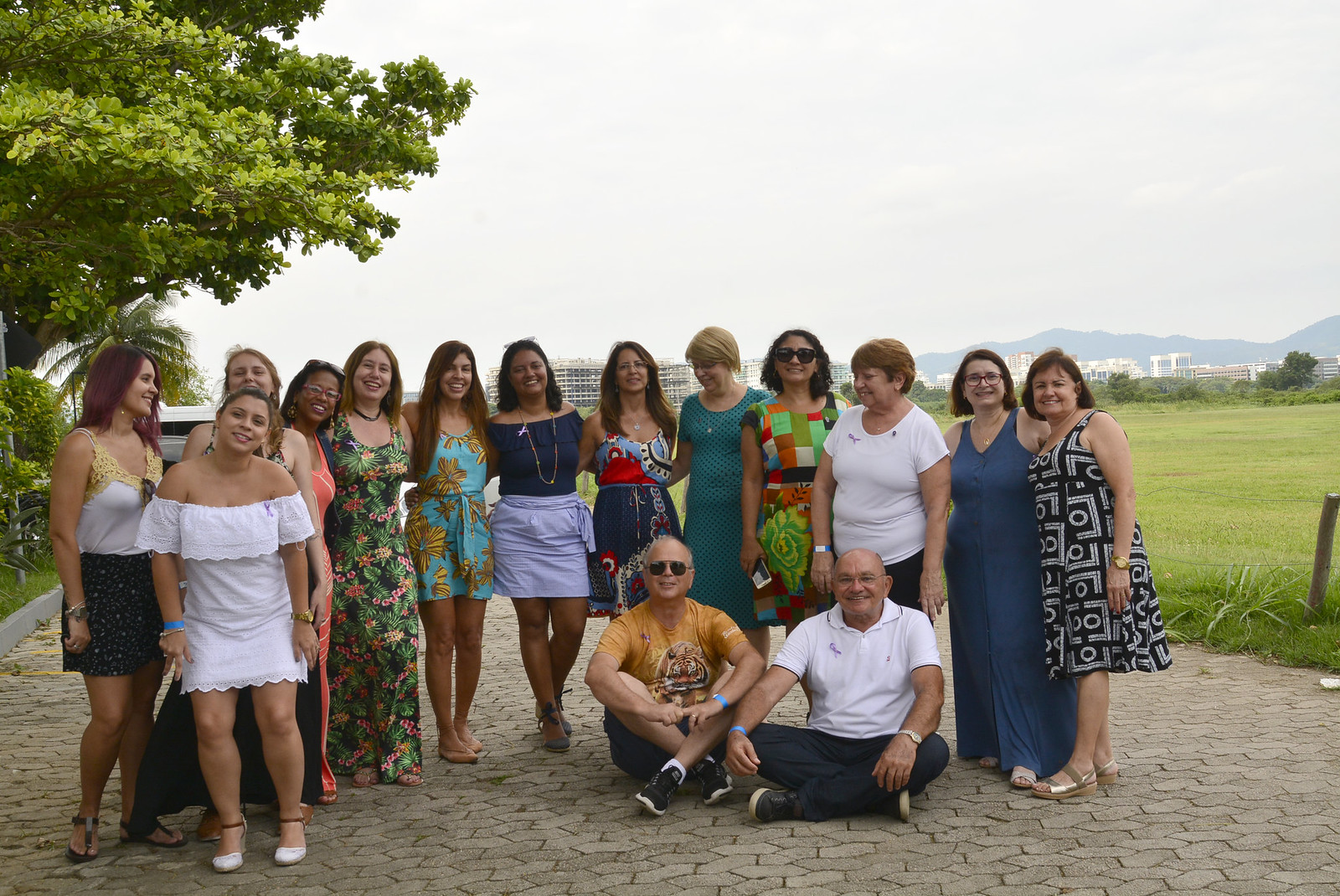A vibrant family reunion captured on a picturesque brick road, with a backdrop of charming buildings and lush green open spaces. Smiling faces abound, with family members adorned in unique, colorful dresses, celebrating their time together under the cool shade of verdant trees. The joyful gathering includes a young woman, 21 years old, who stands out as a beacon of excellence. Her journey reflects a blend of the best attributes from Russian and American cultures, instilled by a mother with high standards. This inspiring young woman is poised for greatness, with aspirations reaching as high as the presidency. The moment is filled with excitement and anticipation as the family enjoys their reunion before parting ways.